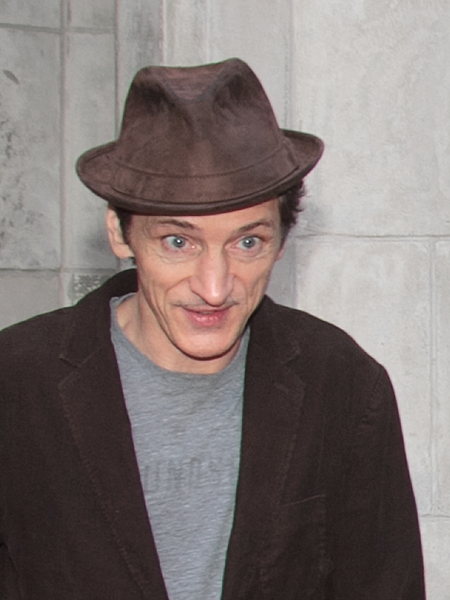The photo features an older white man standing in front of a white wall composed of large brick-like blocks with grayish, somewhat dirty areas. The man, appearing to be in his 40s, sports a distinctive pencil-thin mustache, and his sunken cheeks and wrinkles from his nose down to his chin accentuate his prominent features. His striking blue eyes gaze slightly downward and to the right of the camera. His dark, somewhat curly hair peeks out from underneath a brown felt fedora. He is dressed in a black jacket with a pocket on the front, covering a gray t-shirt that displays partially obscured, faded lettering, including the letters U, N, D, and S.